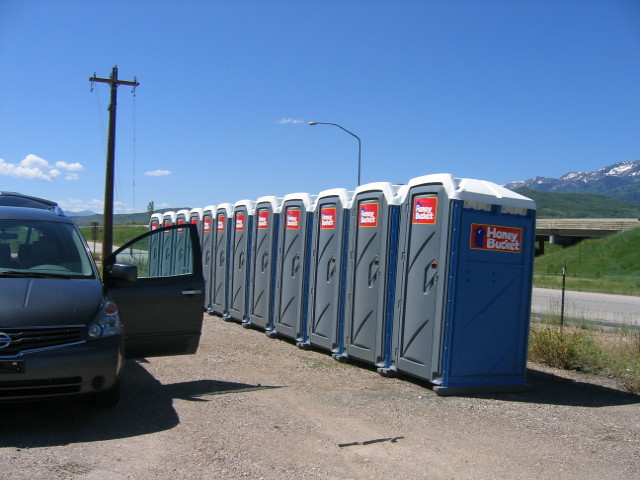The photograph depicts a series of 12 blue port-a-potties lined up along the side of a dirt road. Each port-a-potty features the text "Honey Bucket" displayed prominently on both the front and side, indicating the servicing company. Adjacent to the port-a-potties is a car positioned to the left, with its driver's side door and trunk open, facing the viewer. Further back in the scene, a pole with a power line is visible, and there is another road beyond the port-a-potties. In the background, the clear blue sky is dotted with a few clouds, and towering mountains with patches of snow add a picturesque quality to the otherwise utilitarian scene. The setting suggests a remote or rural area, likely in America, as inferred from the visible highway, overpass, and additional roadside features like a streetlight and the back of a highway sign.